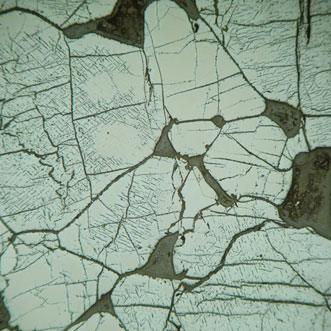This image depicts a fragmented and disordered surface resembling broken tiles. The shattered tiles, in various shapes and sizes, expose the old mortar underneath. The tiles are predominantly off-white with splashes and fractures of blue, gray, and a bluish-green hue, adding to their chaotic appearance. The jagged fractures crisscross the surface, reminiscent of an ancient, apocalyptic ruin or a shattered mosaic. The lack of uniformity and the scattered lines evoke the imagery of a crunched up leaf or a microscopic cell structure, further detailed by the random straight lines that can be likened to roadways or subway lines. The overall visual is akin to an abstract map, filled with intricate and errant patterns that suggest a complex, yet broken architectural past.